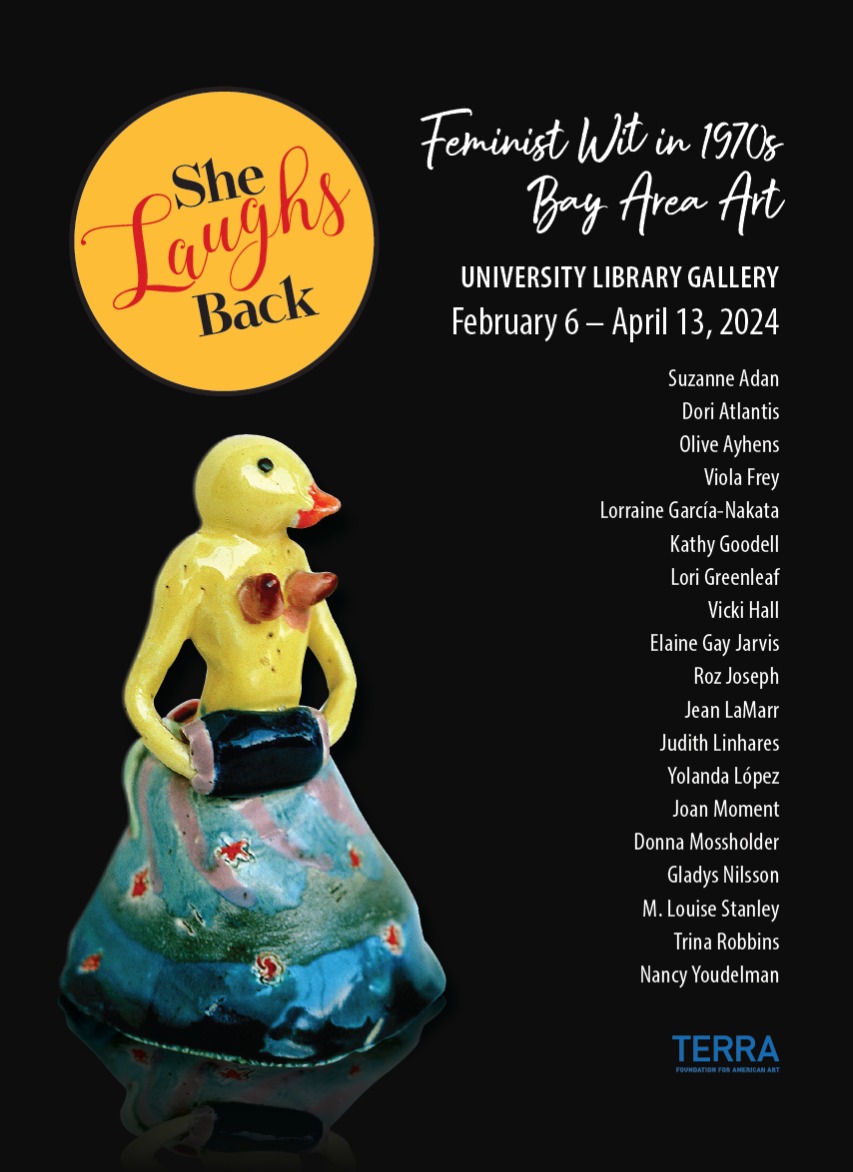This vibrant poster, set against a stark black background, prominently features a yellow circle in the upper left corner with the red cursive text "she laughs back," where the words "she" and "back" are in black. To the right is a column of white text detailing the exhibition title "Feminist Wit in 1970s Bay Area Art" followed by the venue and dates: "University Library Gallery, February 6 - April 13, 2024." It lists the artists' names, such as "Suzanne Adan, Dorri Atlantis, Olive Ahens, Viola Frey, Lorraine Garcia Nakata, Kathy Goodell, Lori Greenleaf, Vicky Hall, Elaine Gay Jarvis, Roz Joseph, Jean Lamar, Judith Lynn Hares, Yolanda Lopez, Joan Moment, Donna Mossholder, Gladys Nilsen, M. Louise Stanley, Trina Robbins, and Nancy Udelman." On the left side of the poster is a whimsical figurine of a yellow duck adorned in a blue dress with red stars, holding a black purse. The bottom right corner features a blue logo with the name "Tara."